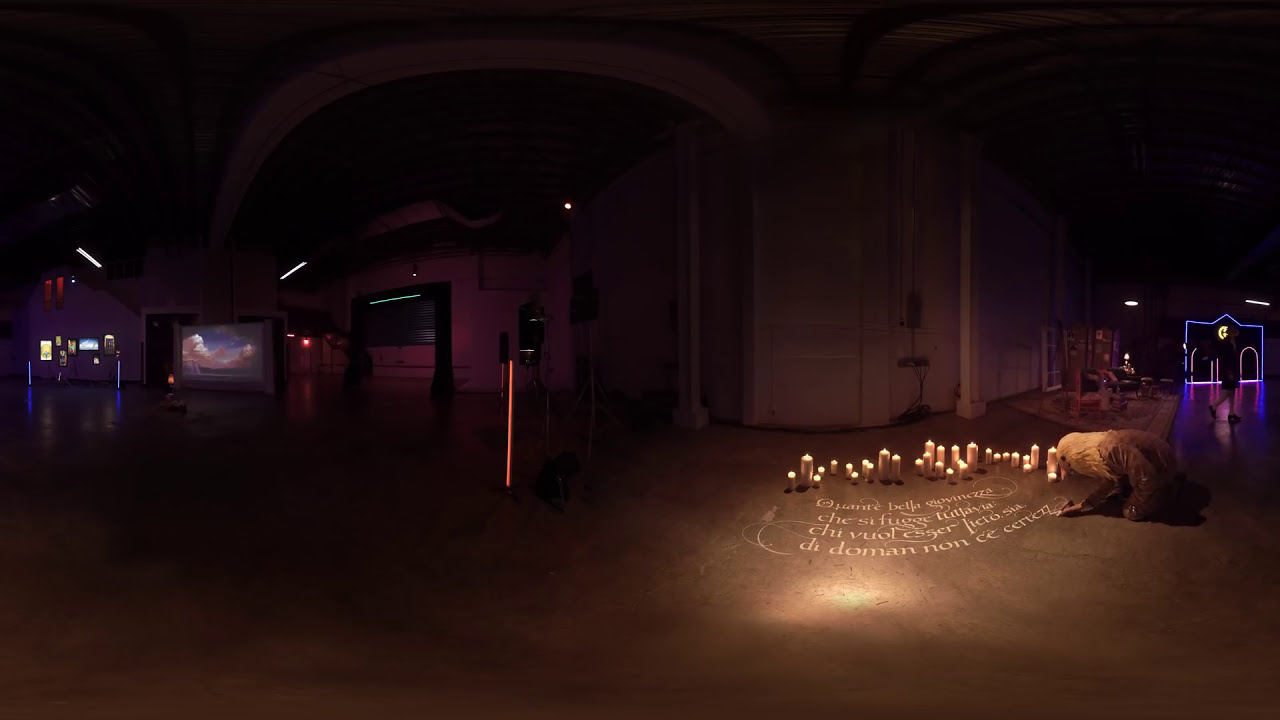The image depicts the interior of a large, dark room with high, curved ceilings adorned with white wooden walls. The room has an artistic, almost abstract ambiance and appears mostly empty. Central to the image, an individual in a hooded cloak, wearing a bird-like mask, is bent over, writing in chalk on the ground in what seems to be Latin or possibly another foreign language. Their elegant, flowing handwriting is framed by a row of lit candles that bathe the scene in a warm glow. To the right of this person, a beautiful Persian rug lies on the floor. The background of the room features various elements, including a set design piece that looks like a neon-outlined house or doorframe and some lit-up projection screens attached to the walls. There are also hints of theater set pieces, including chairs scattered around. The overall lighting in the room is minimal, with the primary sources being the candles, small lights, neon signs, and the projection screens, creating a panoramic and somewhat enigmatic visual experience.